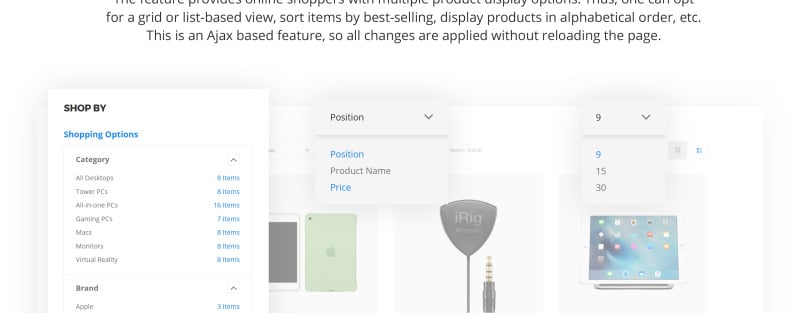This screenshot represents a segment of an e-commerce website, showcasing a product sorting and filtering interface. 

At the top section, a partially visible block of gray text on a white background discusses sorting options for users, such as arranging items by best-selling, displaying products in alphabetical order, and other sorting methods available in a grid or list-based view. It also mentions that these features use Ajax for seamless updates without reloading the page.

To the left, a "Shop By" category is indicated, with "Shopping Options" prominently displayed in blue text. Just below, bold lettering highlights a drop-down menu with various product categories and item counts: 
- All Desktops (8 items)
- Tower PCs (8 items)
- All-in-One PCs (16 items)
- Gaming PCs (7 items)
- Macs (8 items)
- Monitors (8 items)
- Virtual Reality (8 items)

Further down, the "Brand" category lists "Apple" with 3 available items.

To the left of this text is an image depicting a green iPad. To its right, there is a sorting options menu including fields like "Position," "Product Name," and "Price." Adjacent to these fields, there's a reference to a product from a brand called iRig, resembling a US headphone jack.

Below, there's a selection drop-down allowing users to choose how many items to display per page, with options for 9, 15, and 30 items. Beneath this, another image shows an iPad screen populated with default apps, such as Photos, Messaging, and Settings.